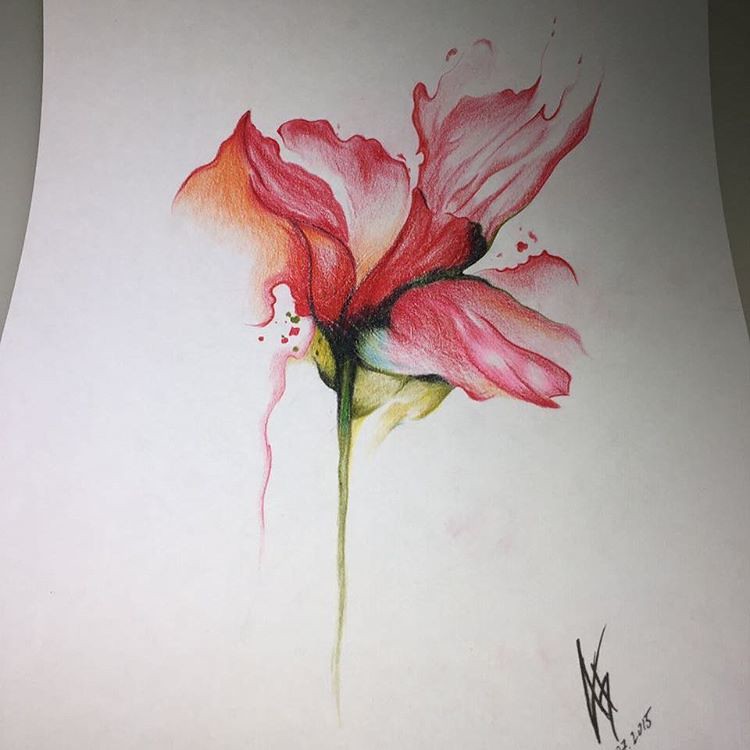This image features a surrealist watercolor painting of an ethereal flower that converges toward the center of the paper. The flower, with its delicate and wispy edges, appears to be blooming open yet remains unfinished. Predominantly rendered in shades of pink, red, and orange, the petals exhibit a gradient of colors, transitioning to warmer hues and incorporating subtle hints of yellow and white. Notably, the left petal remains unfinished, accentuating the fluidity and dreamlike quality of the artwork. The petals also possess a scalloped edge that contributes to their intricate appearance. This fantastical flower is anchored by a dark green stem that tapers off and loses detail towards the bottom. The piece is signed by the artist at the bottom with a date, 3.2015, and shows signs of skillful color manipulation, with pigments seemingly dripping down the page, adding to its whimsical and fluid nature.